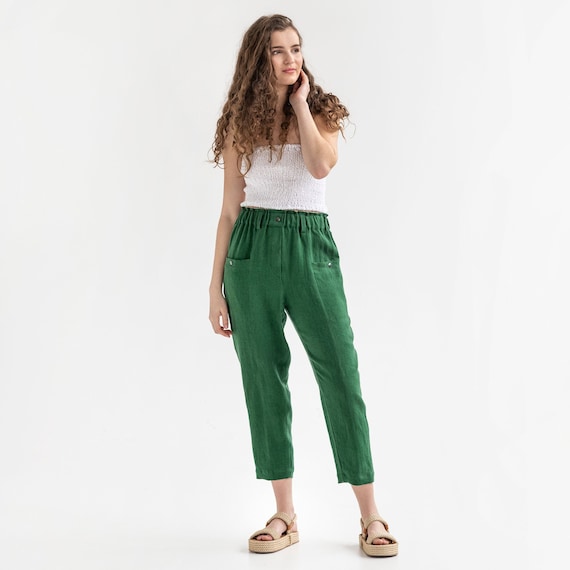This image features a young Caucasian woman posing against a white backdrop, most likely modeling clothing for a fashion advertisement. She has long, curly brown hair and is wearing red lipstick, giving her a striking appearance. Her outfit consists of a white, textured, strapless tube top that has a vintage feel, paired with loose-fitting green pants that have a stretchy waist and fall to mid-calf. The pants, notable for their practical pockets, have two buttons at the waist. On her feet, she wears tan sandals with two-inch platforms, featuring a strap across the toes, another over the top of the foot, and one around the back of the ankle. Her pose is dramatic, with her left hand touching her cheek and her gaze directed off to the left, reminiscent of a professional fashion shoot.